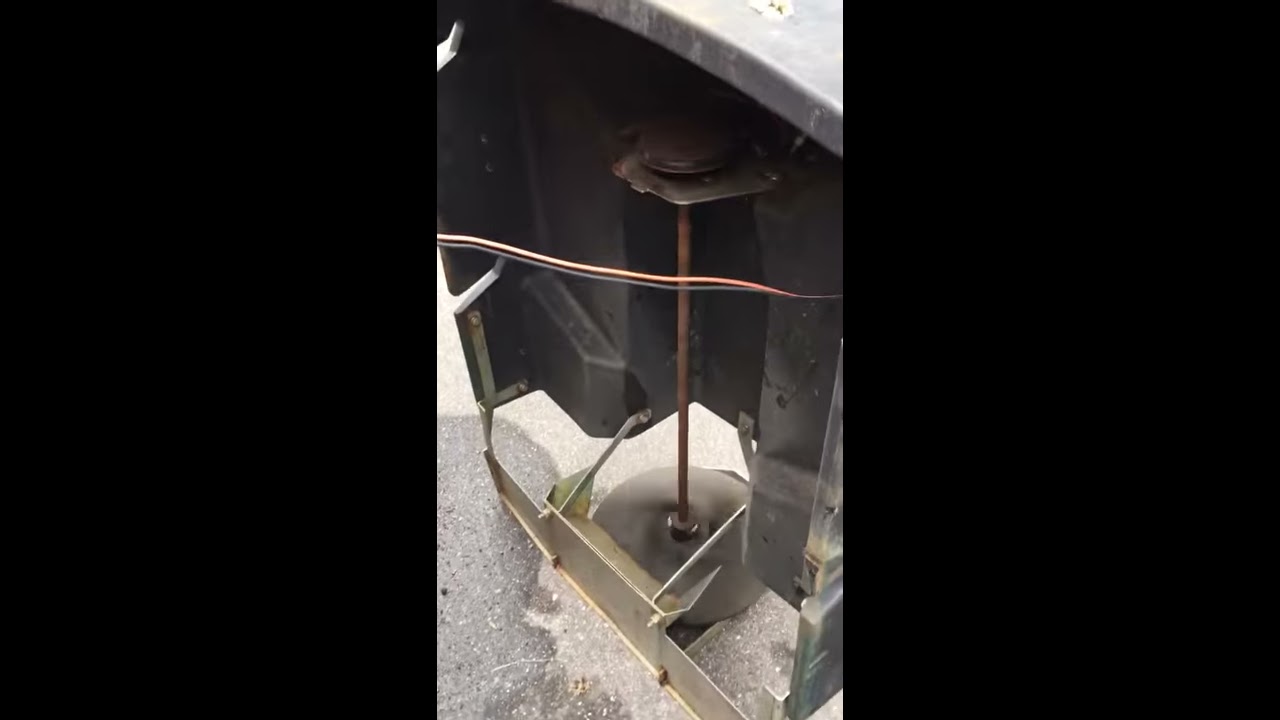The image features an industrial piece of cutting machinery, with a heavily detailed and rust-speckled metallic black case that encloses the central components. The case is secured with numerous bolts and exhibits various rust spots. Inside, a prominent metal rod or axle extends vertically, capped with a small, rusted round top and ending in a large, flat blade that points downward. This blade appears almost pressed against the asphalt ground beneath the machinery. Adjacent to the blade is a brass-colored metal guard, firmly mounted to the device. A red wire is visibly draped across the top of the apparatus from right to left. The surrounding setting includes a concrete or asphalt surface, with hints of shadows cast, possibly from a person standing in front of the machinery. The interior setup also seems to include a silverish metal bracket and clamps that hold the structure together, adding to its complex yet functional industrial design.